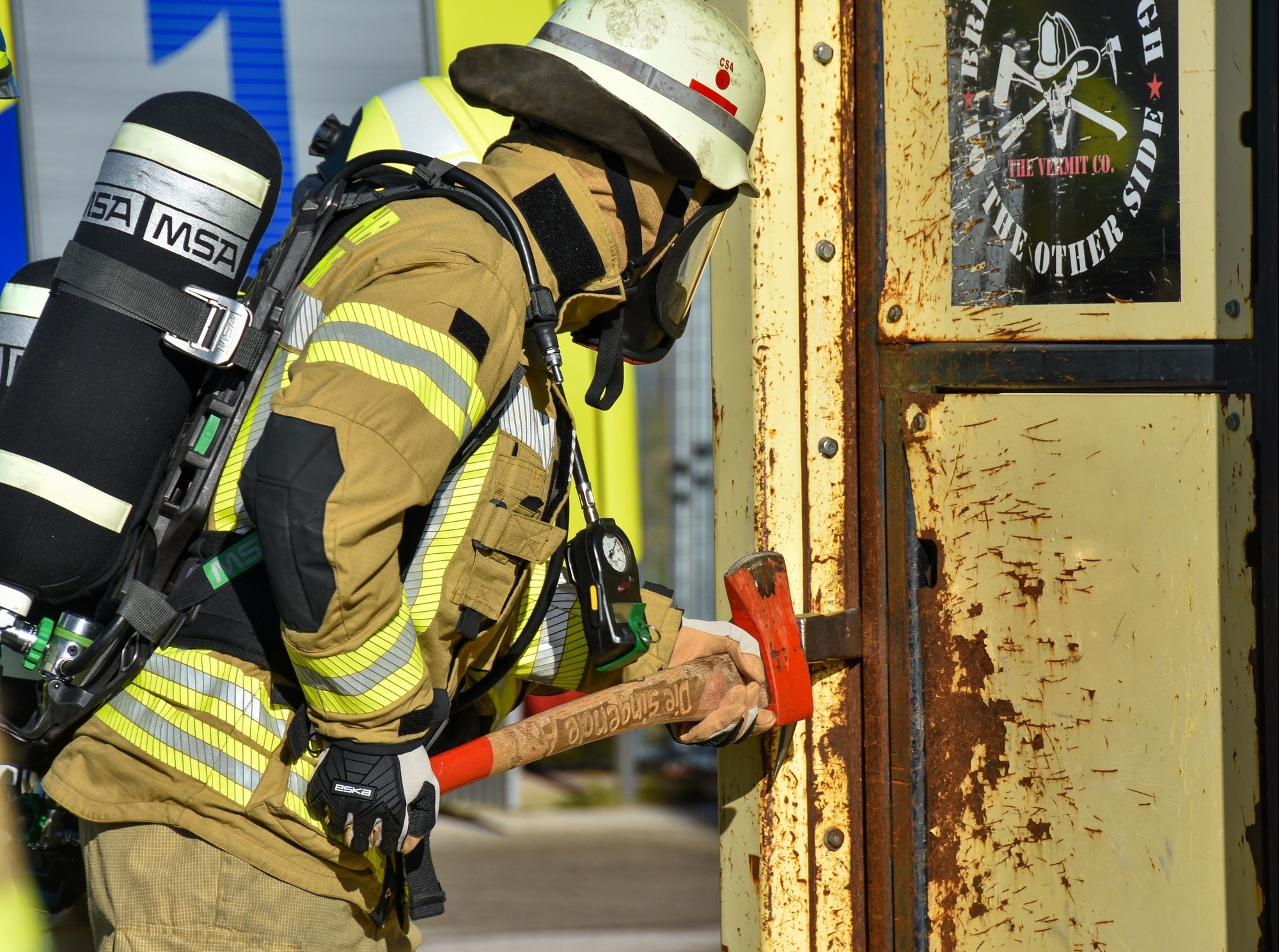In this detailed color photograph captured during daytime in landscape orientation, a fireman fully outfitted in his protective gear is seen performing a drill. The fireman is dressed in a tan firefighter uniform adorned with yellow and silver reflective stripes on his arms, chest, and waist. His protective ensemble includes a white hard hat, a black face mask with a large transparent visor, and a pair of gloves—one black and white, the other brown and white. Strapped to his back is a black breathing air tank.

The fireman is concentrating on a rusted metal door, which is painted yellow and marred with numerous scratches and cuts, indicative of extensive use. This door, studded with numerous rivets, features a skull emblem resembling a fireman with a pick and an axe behind it, and partially visible text related to "vermin company." In his hand, the fireman firmly grips a large axe with a bright red head and handle emblazoned with text that’s difficult to decipher. He is using the flat end of the axe to wedge open the rusted door, not the sharp blade, showcasing his skill and exertion in this training scenario.